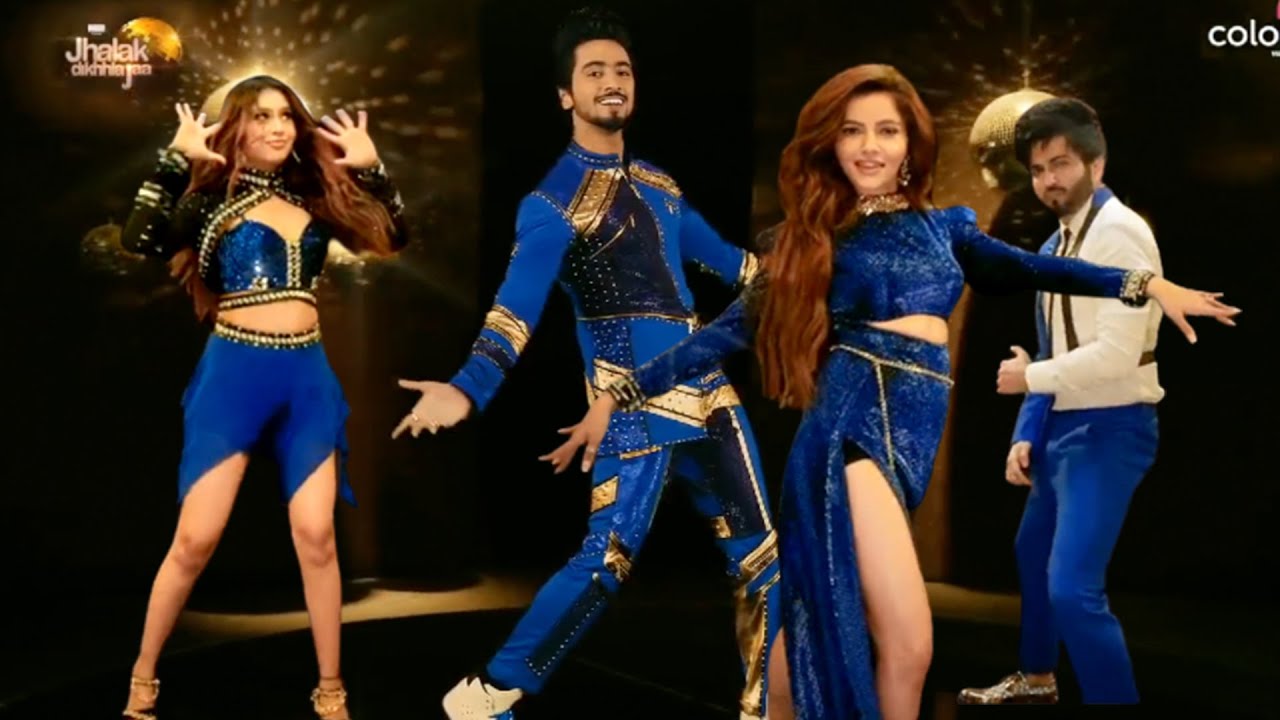The image captures an electrifying action shot of four dynamic performers against a dramatic black backdrop punctuated by gleaming disco balls emitting golden lights. Positioned from left to right, the scene begins with a woman in blue shorts matched with gold sandal-like shoes. Her expressive pose features both hands open, palms outward near her face, and her gaze is directed upwards to the right, embodying a moment of joyous energy. Beside her, a man adorned in a distinctive patchwork dance costume, blending dark blue and gold, strikes a confident stance with his palms facing downward and his left foot extended while smiling radiantly. To his right, a woman exudes sophistication in a dark blue velvet ensemble. Her arms are extended straight out with palms facing down, her right foot leading her poised posture. Completing the quartet is a man in dark blue pants and a striking white shirt featuring a dark blue sleeve on the right. He faces the camera directly, adding a balanced symmetry to the composition with his attentive expression and body angled towards the left. The golden reflections from the disco balls enhance the vibrant, celebratory atmosphere, casting a magical glow over the entire scene.